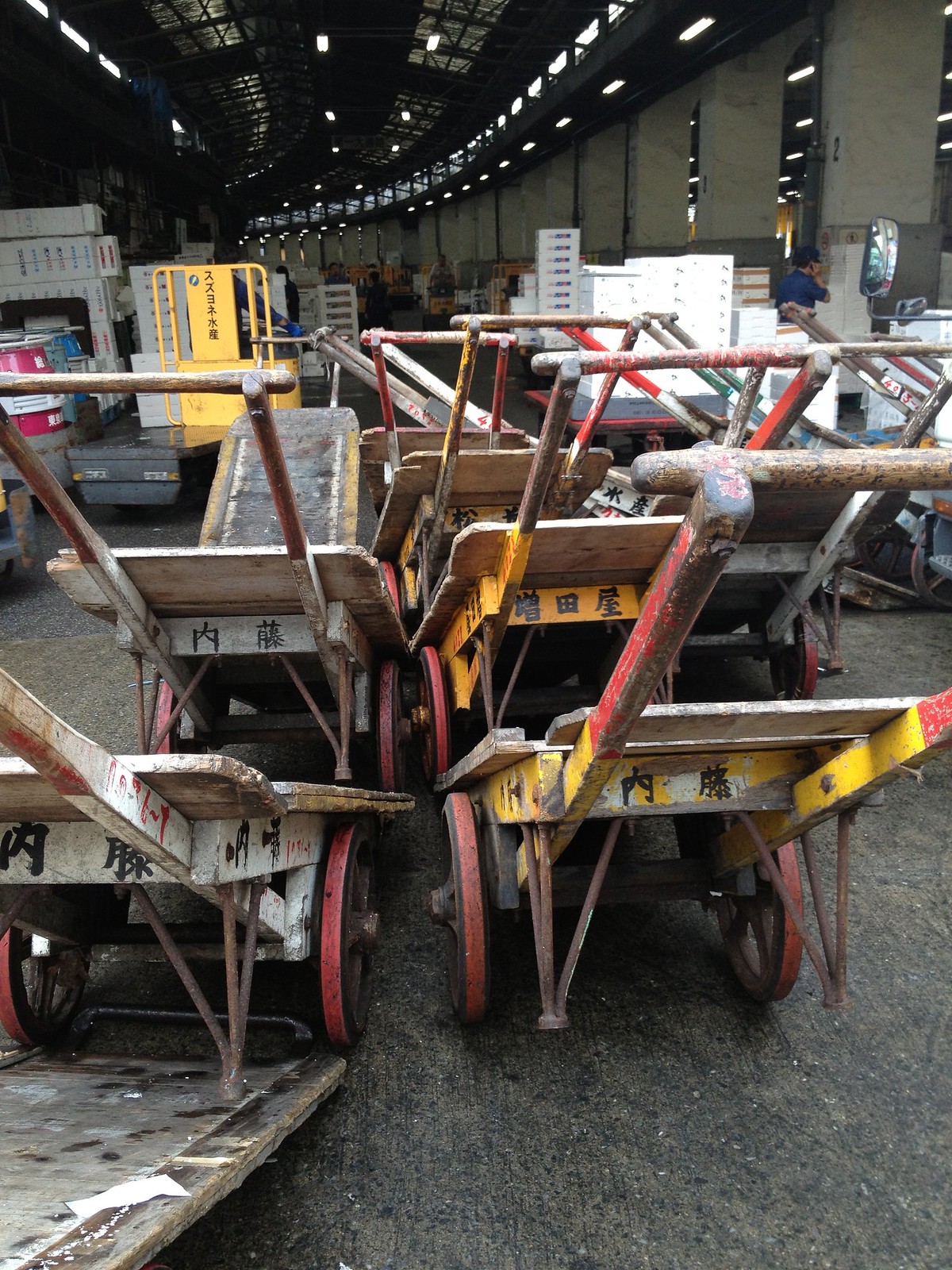This color photograph captures the interior of a bustling warehouse or market in what appears to be an Asian locale, possibly Japan or China. Central to the image is a row of handmade wooden carts with steel wheels and wooden spokes, adorned with Asian characters, likely signifying their purpose or origin. These well-worn, human-powered carts—with their flat platforms painted in hues of red, yellow, and white—are neatly stacked one atop another.

In the foreground, a low ramp extends into the frame from the bottom left corner, guiding the viewer's eye toward the numerous carts lined up for use. The warehouse itself features enormous concrete columns and a ceiling supported by black metal girding, complete with fluorescent or LED lighting, illuminating the vast staging area. This space, filled with various items, boxes, and possibly construction equipment, suggests a bustling environment where goods such as fruits or other market items are regularly loaded and transported. Among the organized chaos, there are individuals in the background, adding to the sense of a busy, operational setting.